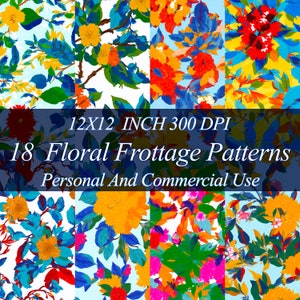This colorful image showcases 18 floral frottage patterns available for personal and commercial use. The patterns are presented in a grid format with 8 visible squares on this particular snapshot, each measuring approximately 1.5 by 1.5 inches, though the full resolution is 12 by 12 inches at 300 DPI. The text, set within a dark band in the center of the image, highlights the size and quality specifications. The patterns display a variety of vibrant colors and floral designs, including light green backgrounds with yellow nasturtiums, white backgrounds with orange and blue flowers, and green leaves. The detailed textures and colors create an appealing and intricate collection of floral patterns suitable for various applications. There is no additional contact or web page information provided in this snapshot.